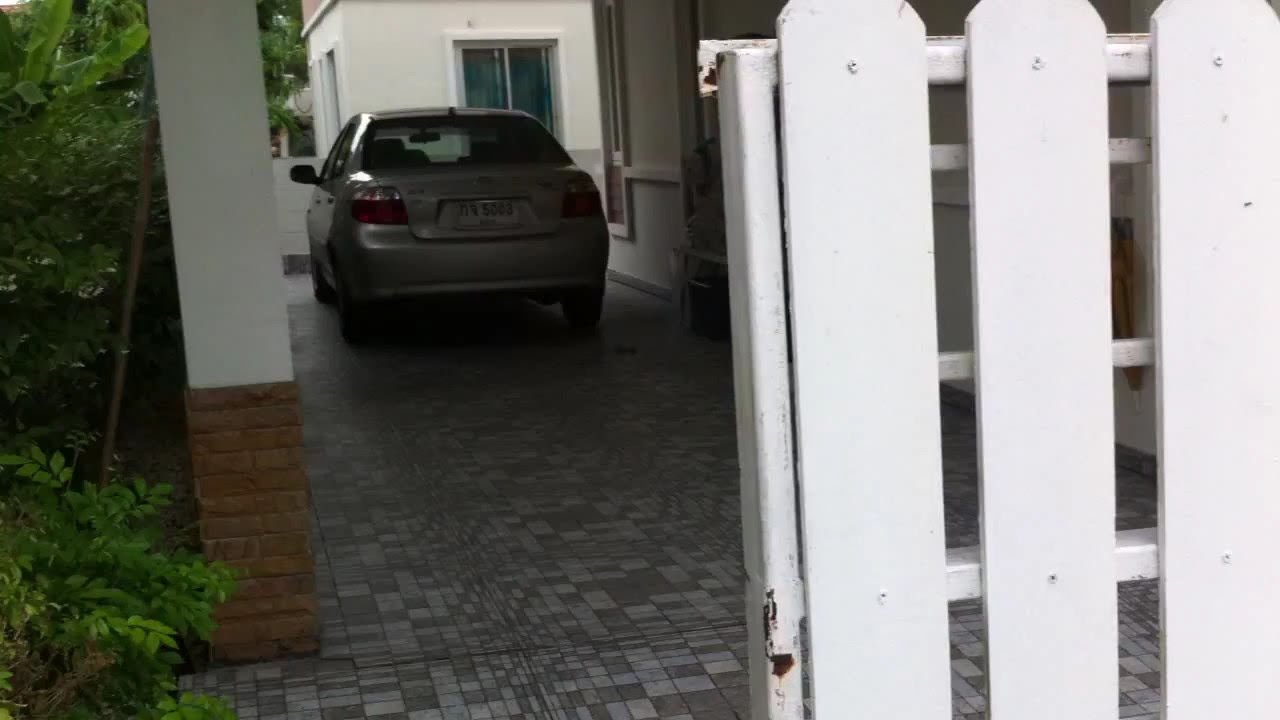In the image, a light-colored sedan is seen parked in a tiled driveway, which consists of small white and gray tiles, just outside a house. The rear end of the car, featuring red taillights and a barely discernible license plate numbered '5003,' is positioned under a white awning held up by white pillars. The house in the background is predominantly white with visible windows and a main entrance ahead of the car. To the left of the car, lush greenery comprising both short bushes and taller trees contrasts with a white and brown cement wall. On the right side of the image, part of a white gate stands open, offering a glimpse of a garden area alongside the parking space. The overall scene emanates a serene, orderly outdoor setting attached to a well-maintained home.